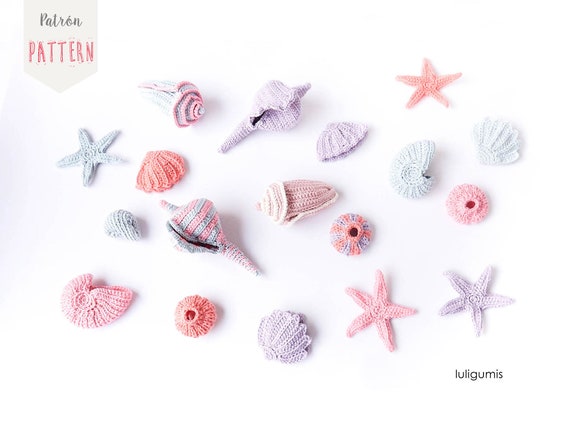This vibrant color photograph features an assortment of intricately crocheted seashells and starfish arranged against an off-white, light gray background. The variety includes approximately 15 items in an array of colors such as pink, blue, salmon, and combinations thereof. Among the seashells are various shapes, including circular, flat, and cone-like forms, as well as four distinct starfish. There's also a unique seashell with a button-like center hole. On closer inspection, the upper left corner of the image shows a small tag or a piece of curled paper labeled "patron pattern" in salmon-colored text, while the bottom right corner features the name "Luligumus" in simple black type. The overall composition highlights the intricate craftsmanship and vibrant diversity of the crocheted pieces.